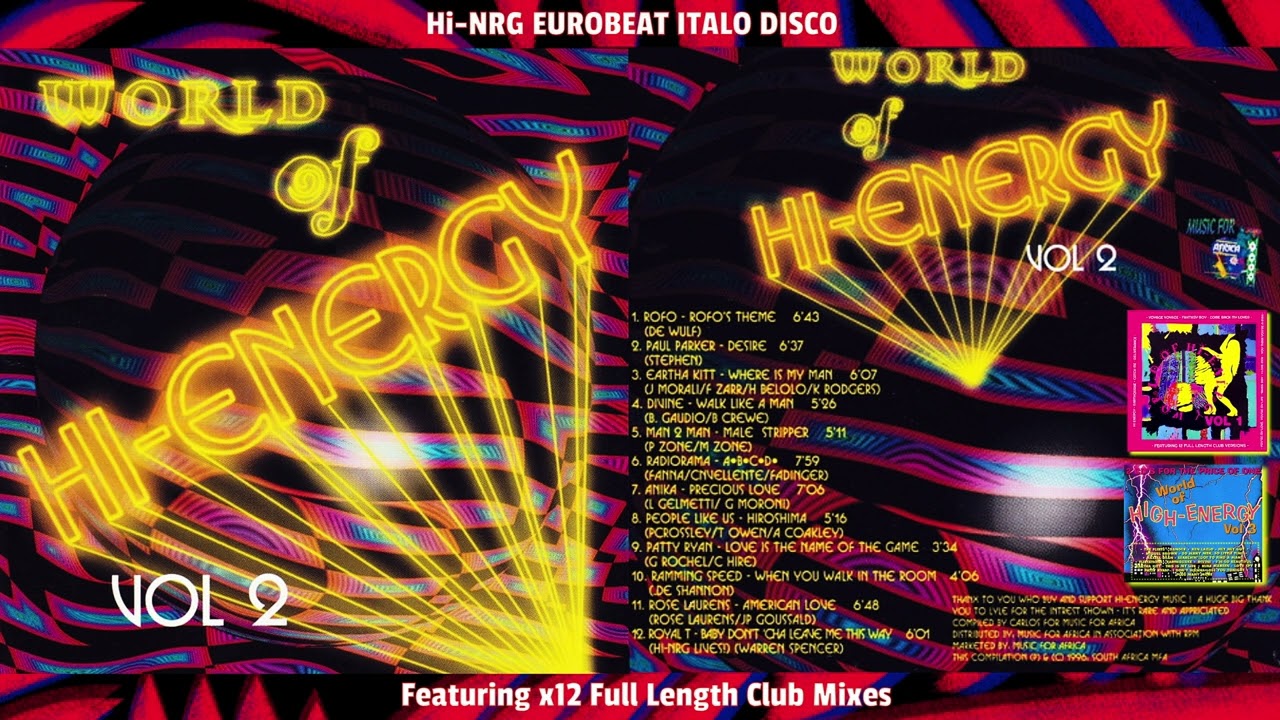The image displays a vibrant brochure or ad print resembling a record cover for an event. It prominently features text written in glowing yellow neon lights. Dominating the left side, the text declares "World of High Energy," further accentuated by "Volume 2" at the bottom. Centrally, the words "High Energy Eurobeat Italo Disco" capture attention. The right side also repeats "World of High Energy," beneath which is a list of songs comprising the album cover. Additionally, there are two rectangular shapes on the right side containing illustrations. The bottom of the image spotlights the text "Featuring X-12 Full-Length Club Mixes." The background bursts with dynamic colors in red, blue, purple, and yellow, accompanied by swirling and lined patterns that enhance the energetic theme.